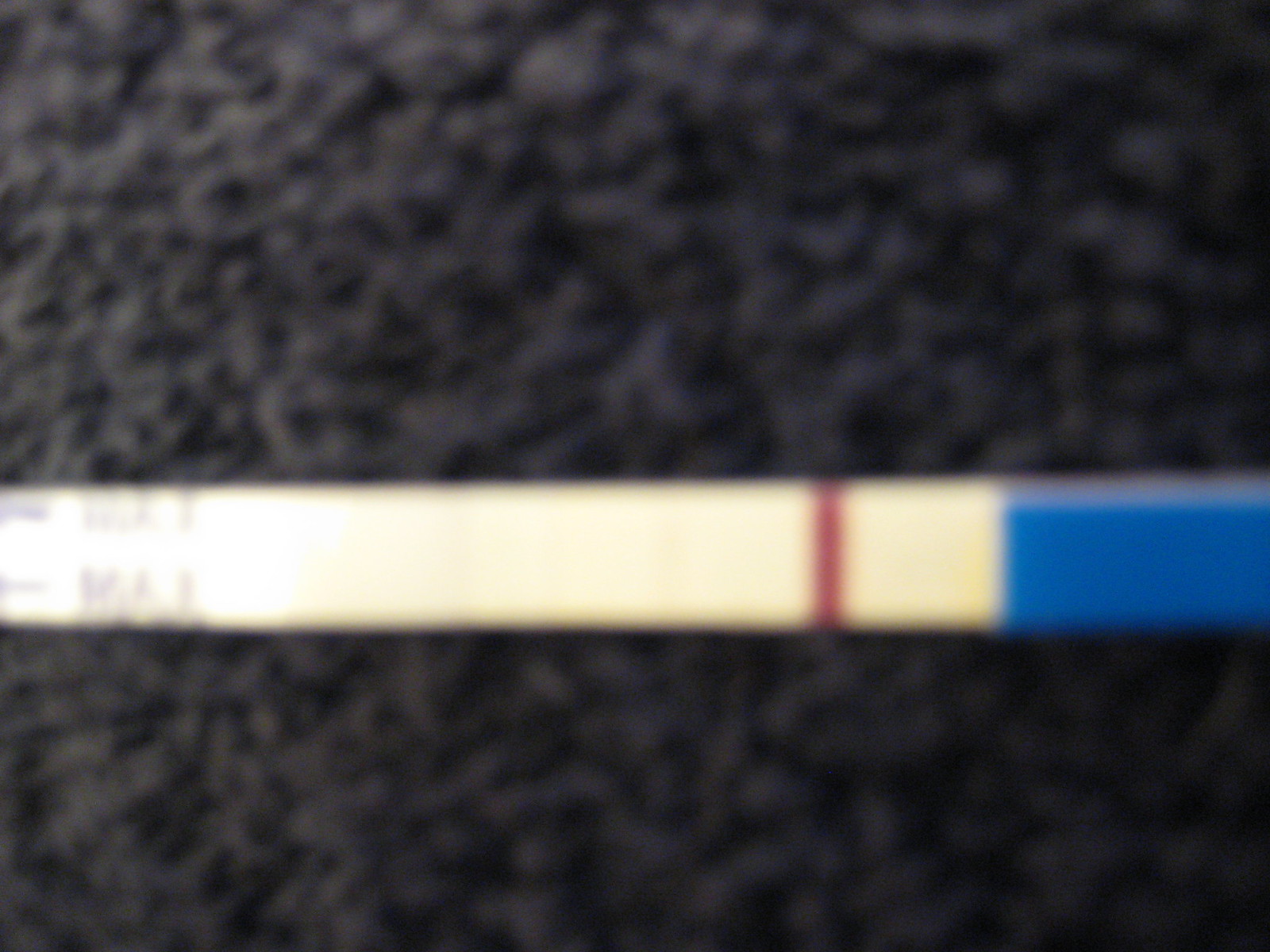The image is a close-up, though slightly blurry, of a beige-colored testing strip. On the left side of the strip, there are several vertical black lines, both along the edge and slightly above the strip. On the right side, a single red line is visible towards the middle of the strip. Additionally, there is a blue square strip situated on the right side. The background features a bumpy black texture, which adds contrast to the focus on the testing strip.